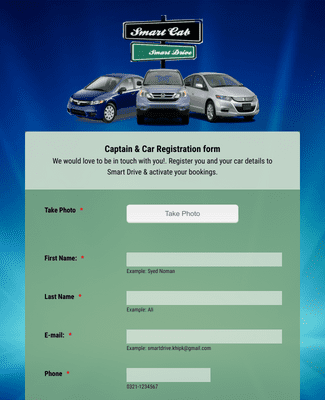This image appears to be an advertisement for Smart Cars. It prominently features a road sign, divided into two sections. The top section of the sign is black and displays the text "Smart Cars" in bold letters. The bottom section of the sign is green and contains additional text, although it is less legible in the description provided.

In front of the sign, there are three Smart Cars displayed. Below the cars, there is text that appears to read "captain and car registration form." The advertisement encourages viewers to register their car details with the Smart Drive program, offering a welcoming invitation with phrases such as "We would love to be in touch with you" and "register you and your car details to Smart and Smart Drive."

Part of the form includes instructions such as "activate you for keys" and prompts users to "Take photo." Further, it asks for personal information like first name, last name, and email address.

The background of the image is illuminated with lights, enhancing the overall visual appeal of the advertisement. This implies a modern, inviting atmosphere as part of the Smart Cars branding effort.